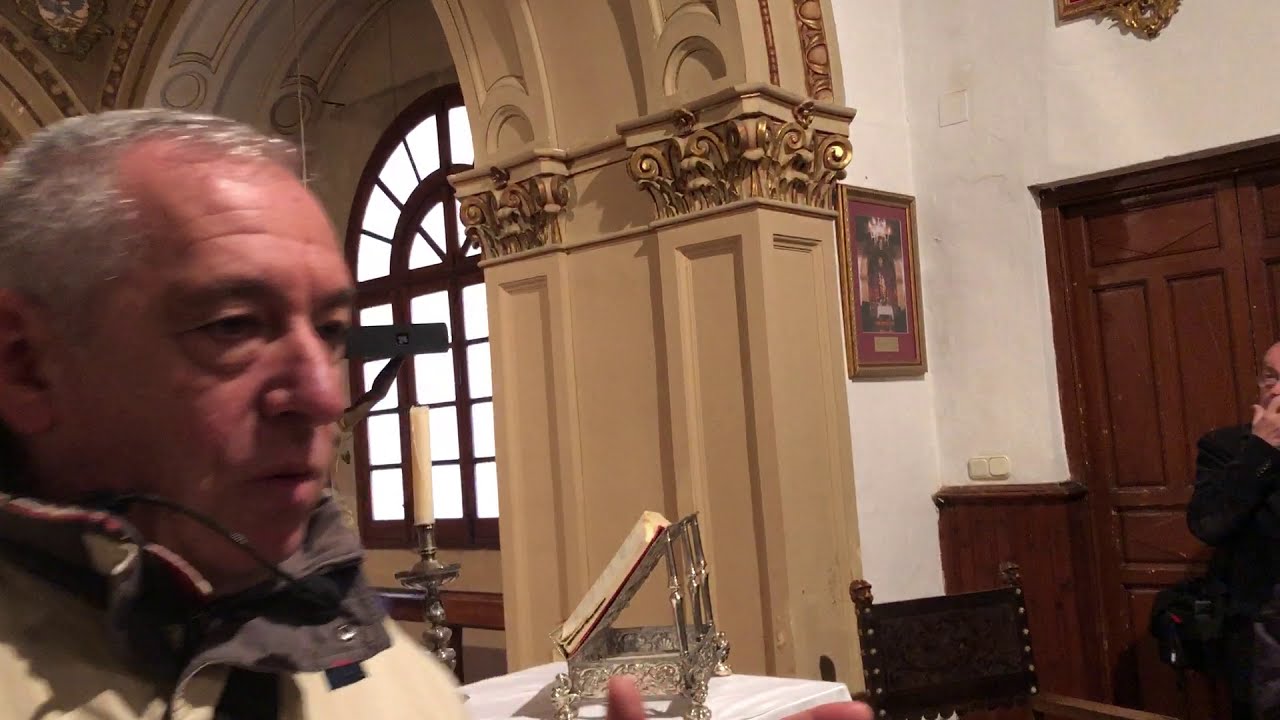This is a photograph of an older man, possibly in his late 50s or 60s, with grey, slightly balding hair, standing inside an elegant and historical building, which might be a church or a museum. The man is positioned in the lower left corner of the image, wearing a winter jacket and appears to have a microphone attached to him. Behind him on a table, there's a tall candle and an elaborate silver pedestal likely holding a Bible. A column with intricate architecture and large windows are also visible in the background, contributing to the building's ornate design. The walls are adorned with pictures, and the lighting suggests it is the middle of the day. In the lower right corner of the photograph, partially cut off, is a woman who appears to be looking at the man. She is wearing black and has glasses. The overall color scheme includes shades of grey, tan, brown, pink, red, black, white, and gold, enhancing the rich, historical ambiance of the setting.